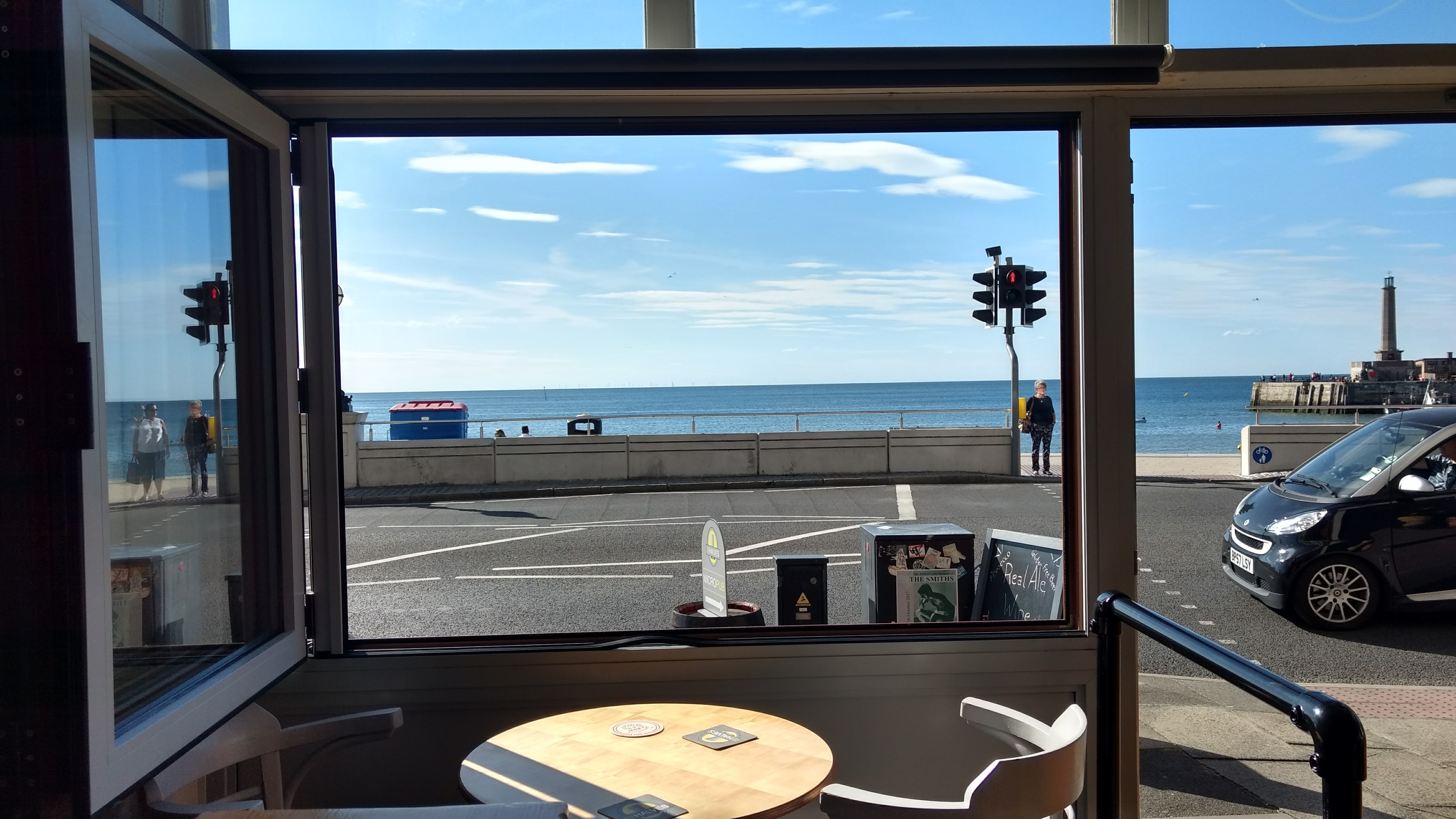The photograph captures a cozy seaside restaurant with a large inward-opening window framing a charming scene. Inside the restaurant, a light brown, round table with two chairs is positioned right by the open window, inviting the ocean breeze to flow in. Beyond the window lies a pavement parking lot, bordered by a low concrete wall with an opening that reveals the sandy beach on the right. The vast blue ocean and a slightly clouded blue sky form a stunning backdrop. In the distance, two swimmers are visible in the water, their heads barely noticeable. A compact, black import car is coming into view on the right-hand side, traveling west. The scene also includes a street light with a crosswalk and the faint reflection of a couple of people in the open window, hinting at the hustle and bustle outside. The setting suggests a serene spot to sit, chat, and enjoy the ocean view, though the parking lot slightly detracts from the otherwise picturesque scene.